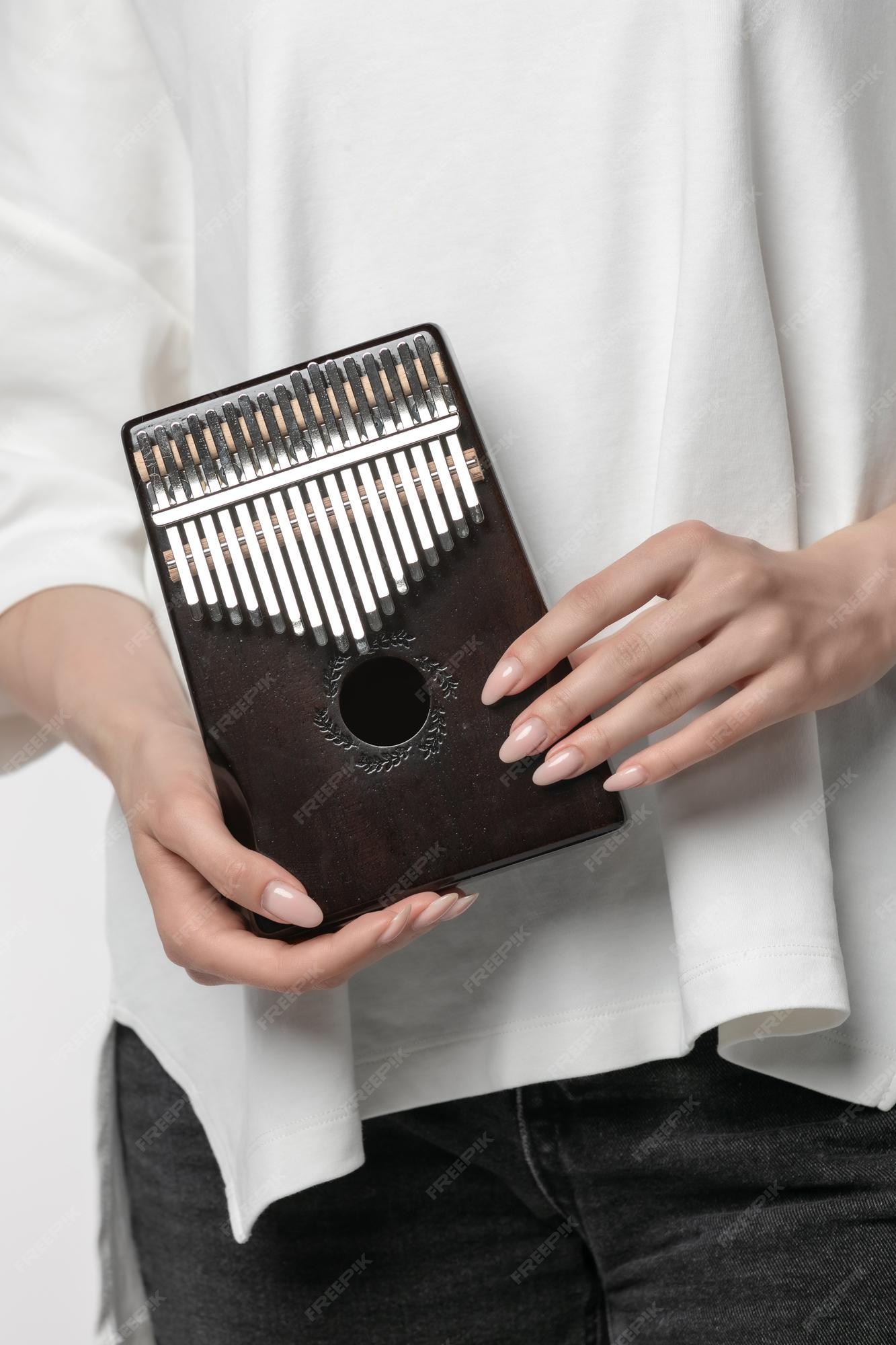The image depicts the mid-torso of a Caucasian woman, identified by her long, nude-painted fingernails. She is dressed in a long, flowing white blouse with three-quarter sleeves and black jeans. The woman is holding a small African musical instrument known as a kalimba, which is roughly the size of a tablet. The kalimba is made of deep, rich brown wood, possibly teak or mahogany, and features a prominent sound hole in the middle. It has about 16 metal tines or keys, which are white with black tips and resemble matchsticks or miniature piano keys. These keys are arranged with the longest in the middle, gradually becoming shorter towards the sides. The woman’s light-colored fingernails and the detailed exotic wood of the kalimba add a contrasting delicate touch to the overall aesthetic of the image, emphasizing the cultural uniqueness of the instrument she is holding.